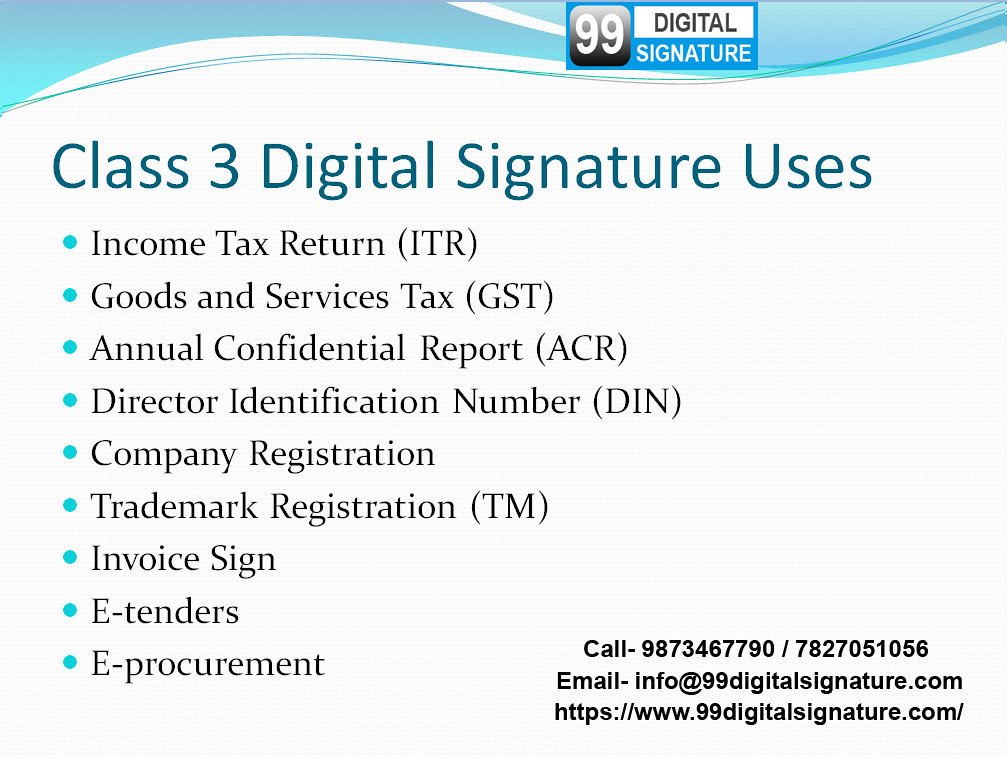This image, likely part of a larger marketing presentation or brochure, features a prominent title in dark blue font at the top center, reading "Class III Digital Signature Uses" above a series of blue and white intertwined curved lines. Featured below the header, a rectangular label displays the number "99" in white, accompanied by the text "DIGITAL SIGNATURE" where "DIGITAL" is in bold black uppercase letters against a white background, and "SIGNATURE" is in white uppercase letters against a blue background. The detailed list below highlights nine uses for Class III digital signatures, each bullet point marked in light blue, and followed by black text:

1. Income Tax Return (ITR)
2. Goods and Services Tax (GST)
3. Annual Confidential Reports (ACR)
4. Director Identification Number (DIN)
5. Company Registration
6. Trademark Registration (TM)
7. Invoice Sign
8. e-Tenders
9. e-Procurements

At the bottom right corner are contact details in black text: "Call 987-346-7790/7827-051056" alongside the email address "info@99digitalsignature.com" and the website "https://www.99digitalsignature.com/".